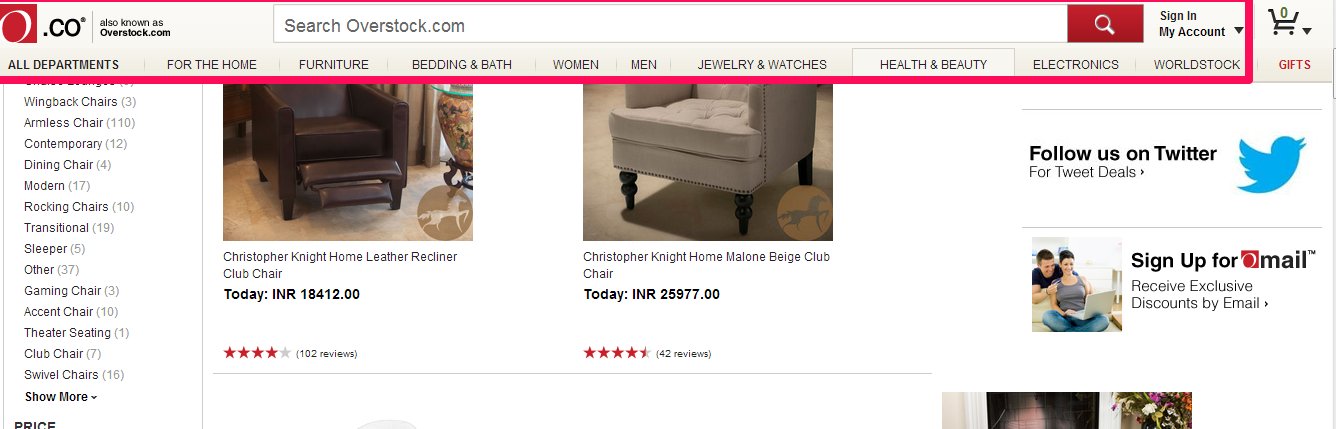Screenshot of Overstock.com furniture section showcasing various categories such as 'For the Home,' 'Furniture,' 'Bed and Bath,' 'Women,' 'Men,' 'Jewelry and Watches,' 'Health and Beauty,' 'Electronics,' and 'World Stock.' Featured prominently is a partial view of several chairs, including a leather and a cloth chair, each with displayed prices and star ratings ranging from 2 to 5 stars. The left sidebar lists approximately 20 different types of chairs along with the quantity available for each type. Ads for social media followership, a shopping cart icon, and a search bar are also visible on the page.